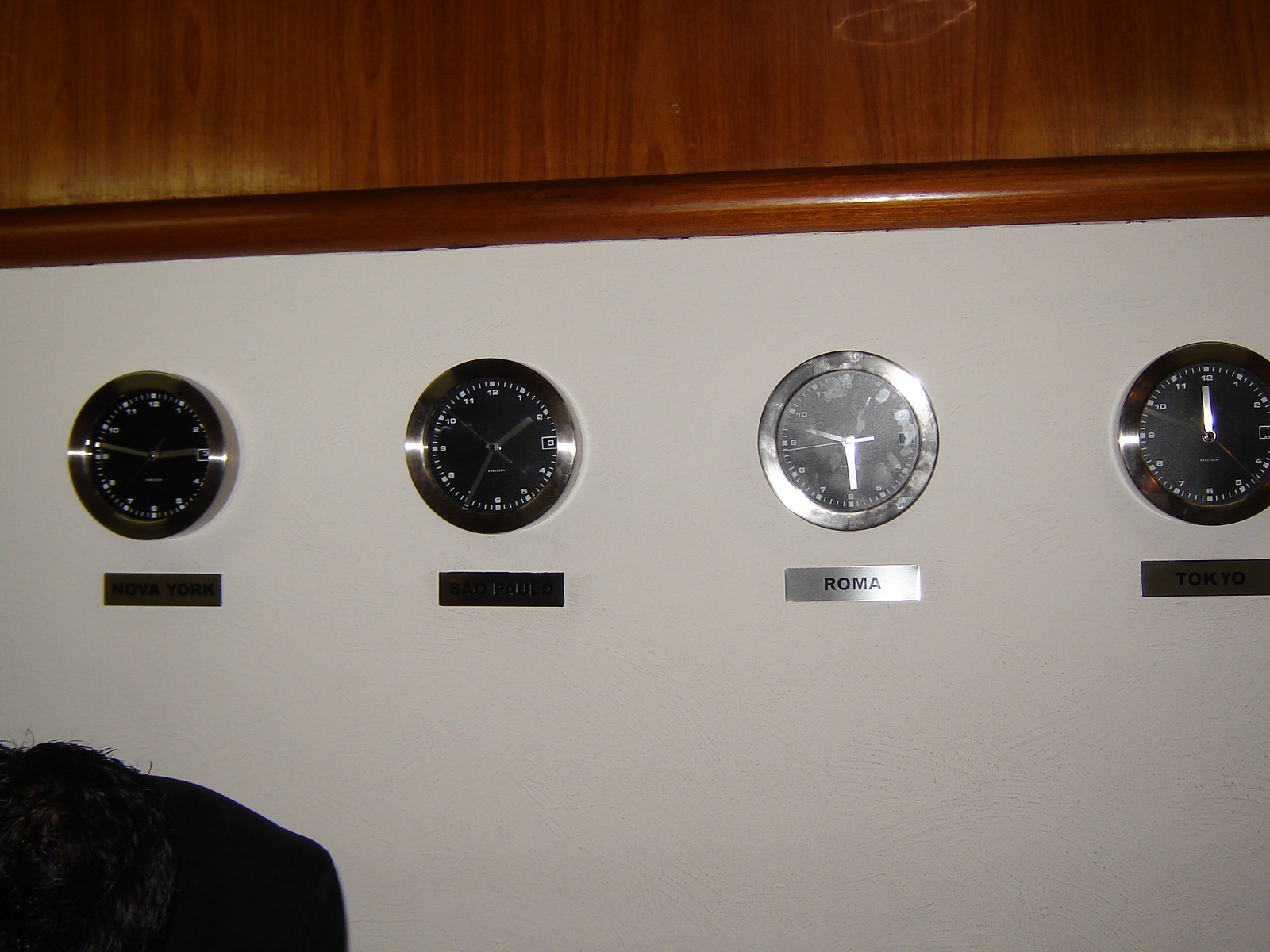This color photograph showcases four round clocks mounted on a white background beneath a paneled wall with a brown wood trim. Each clock has a metallic plaque below it, but only the third from the left has a readable label, which says "Roma." The Roma clock, catching the light and appearing silver with smudges, displays the time with its hour hand roughly at six and its minute hand at about ten. The other three clocks are shrouded in shadow, making the numbers difficult to see, and their plaques unreadable. There is a black smudge or shadow in the bottom left corner of the image. All clocks have plain white numbers from 1 to 12 and minute markers. The white wall below the paneled section has a visible lip or rim separating the two sections.